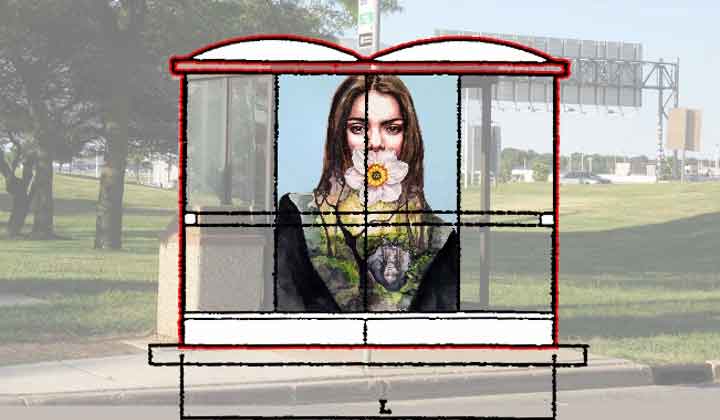The image depicts a creative composition combining a digitally altered photograph of a daytime public rest stop with an illustrative sketch overlay. In the background, a semi-faded scene showcases elements like a bus stop, a trash can, grassy fields, and trees under a blue sky. Prominently, a blurred highway sign and utility pole can be seen blending into the setting. Central to the image is an illustration of a girl with long brown hair and reddish skin, her lips concealed by a white flower with a yellow center. She appears to be wearing a black dress, with a depiction of a forest featuring trees, rocks, and moss on her chest. This figure is set within sketchy black lines bordered by red, creating a striking contrast to the muted tones of the surrounding real-world scene.